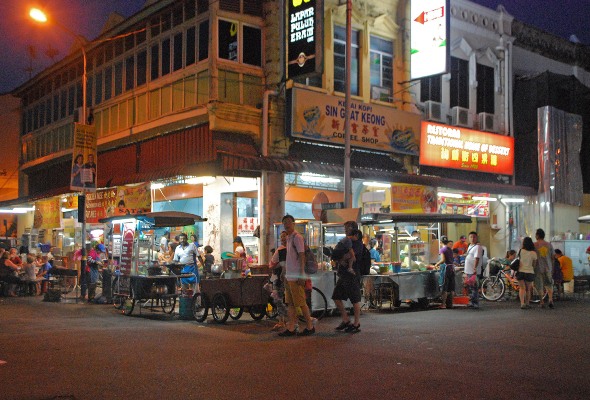This image captures the vibrant atmosphere of a bustling nighttime street food fair in a city that is likely in China. The dark sky and illuminated streetlights enhance the vibrant glow of various colorful signs displayed on city buildings, featuring Chinese characters in hues of blue, yellow, and red. The street is devoid of cars but brimming with life as a multitude of Asian people meander among the numerous food vendors’ carts and tables. These vendors line the sidewalks and corners, offering a diverse array of foods, some employing large griddles and cases, perhaps for frying or popping corn. Among the crowd, a man in a purple shirt is seen serving food, while another man is tenderly holding a sleeping child who rests his head on the man's shoulder. Bicycles are interspersed among the throng of pedestrians, further depicting the lively, yet cozy night scene of the city's bustling street fair.